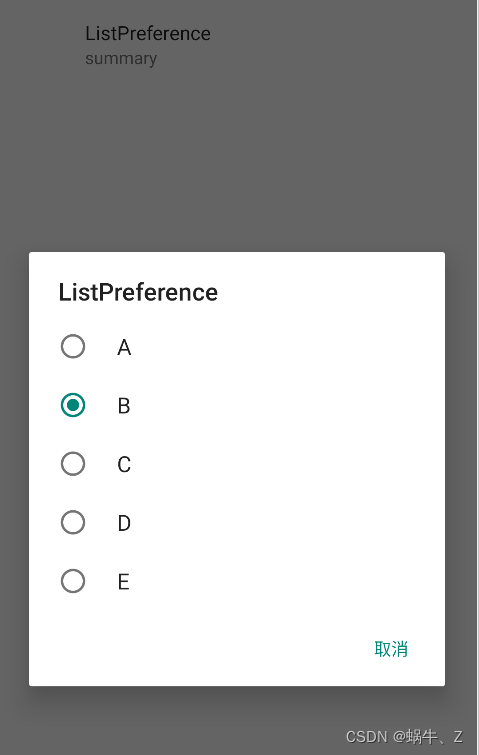The image is a simple screenshot featuring a predominantly medium gray background. Near the top, slightly left of center, black text reads "List Preferences," with "Summary" directly beneath it. Below this heading, there is a horizontally oriented rectangular white box that spans most of the screen width. The white box has a thicker gray border at the top compared to the bottom. 

Inside the white section, the term "List Preferences" is once again displayed, accompanied by a column of bubbles labeled A, B, C, D, and E, where bubble B is selected. An unidentified Chinese character in medium teal is located in the lower right corner of the white section.

Additionally, at the bottom-right corner of the gray border surrounding the white box, the text "CSDN" is displayed, followed by an "@" symbol and more Chinese characters. This intricate arrangement adds context to the otherwise straightforward layout.